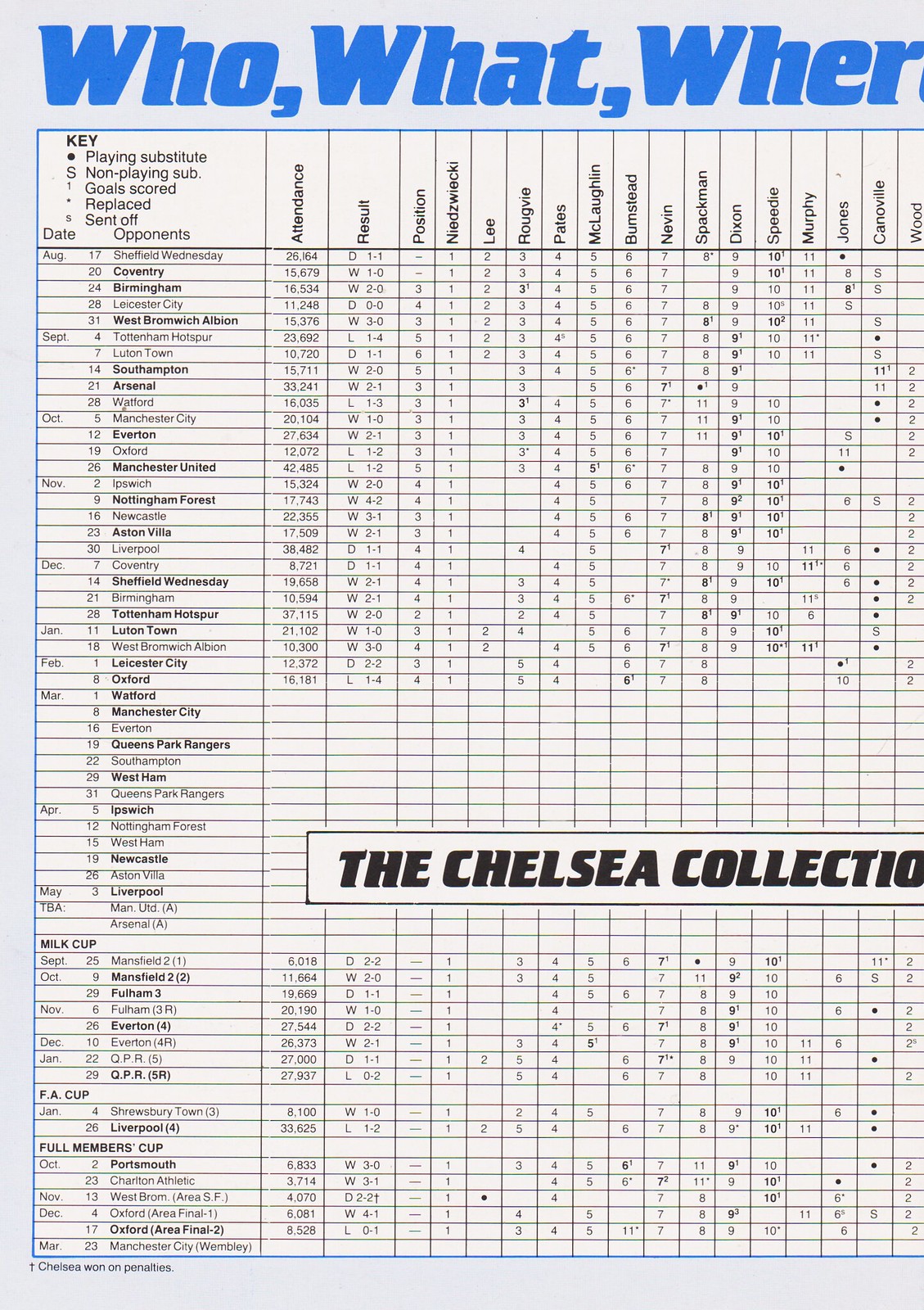This image is a detailed spreadsheet, reminiscent of an Excel sheet, for a soccer club in England, specifically Chelsea. The top of the spreadsheet prominently features big blue text that reads "who, what, where," though the "e" in "where" appears cut off. The spreadsheet itself is white with black text, creating a clean and typical appearance.

A key in the top left corner denotes symbols for playing substitute, non-playing substitute, goal scored, replaced, and sent off. The far-left column lists dates formatted by month and day, and the next column lists opponents, some in bold possibly to indicate home or away games. The attendance column, written vertically, includes figures mostly in tens of thousands, though some entries are in single thousands. The result column indicates outcomes with D (draw), W (win), or L (loss) and the corresponding scores. The position column isn't clearly explained but could refer to player positions or team standings.

Individual player names are given their own columns, with each row corresponding to a date and opponent. These players include Niedzwiecki, Lee, Rougvie, Pate, McLaughlin, Bumstead, Nevin, Spackman, Dixon, Speedie, Murphy, Jones, Canoville, and Wood. Each player's column is populated with corresponding numbers for each match entry.

Additionally, there is bold text stating "The Chelsea Collection" centered near the bottom third of the spreadsheet. Below this, the schedule is broken down by competition: from August to May with "TBA" for unannounced fixtures, the Milk Cup (September to January), the FA Cup (January), and the Full Members Cup (October to March). Each section maintains the same structure of attendance, results, positions, and player data.

Overall, the spreadsheet encapsulates comprehensive match and player data for Chelsea FC, organized in a structured and clear format with a blue border around the entire page.